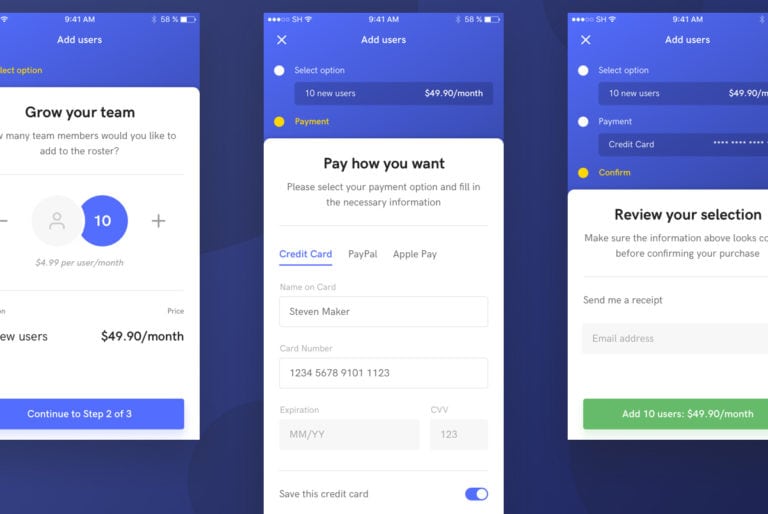This image illustrates three sequential screenshots of a phone interface, displaying the process of adding new users to a service plan. 

In the first screenshot, the top of the screen features a blue header with the text "Add Users." The phone's status bar indicates a battery level of 68% and a strong signal. Below the header, the screen presents a white background with the message "Grow your team. Many team members would like to add to the roster." It includes a plus and minus sign for adjusting the number of users. There is a round profile icon and a blue circle with the number 10, indicating the addition of 10 new users at a rate of $4.99 per user per month. The total monthly charge shown is $49.90, suggesting that the user currently has some subscribers already. A prompt at the bottom reads "Continue to step 2 of 3."

In the second screenshot, the process proceeds to the payment stage, highlighted with a yellow header indicating "10 new users, $49.90." The screen instructs the user to "Please select your payment option and fill in the necessary information." Options for payment include "Credit Card," "PayPal," and "Apple Pay," with "Credit Card" being underlined in blue, indicating it as the selected option. The user details shown include the name "Steve Maker," card number, expiration date, CVV number, and an option to save the credit card information, which is turned on.

The third screenshot confirms the choices made in the previous steps. The screen reiterates "Add Users, Select Option," and "10 new users, $49.90 a month," followed by the payment method "Credit Card." A prominent yellow circle at the bottom of the screen features the word "Confirm," prompting the user to finalize their transaction.